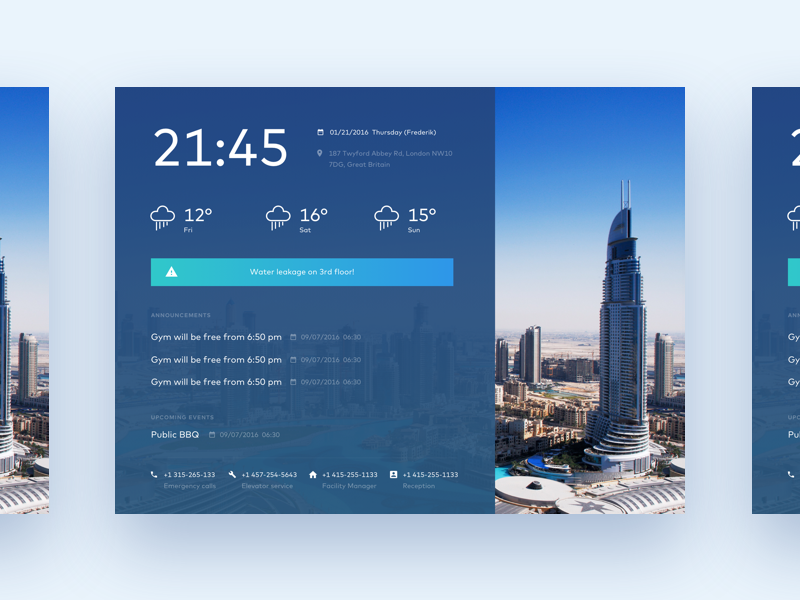This appears to be a screenshot from a weather application, likely taken on a phone, despite its resemblance to a desktop view. The image details the weather forecast for Frankfort on January 21, 2016, a Thursday at 9:45 PM (21:45 in 24-hour format). It was a cold night with temperatures recorded at 12 degrees. The forecast for the following days predicted 16 degrees and 15 degrees, with rain expected each day. Despite the cold and rainy forecast, the current image shows a scenic cityscape under a picturesque blue sky.

Additionally, the image indicates that "Jim" will be free from 6:50 PM onwards for three consecutive days. There is a mention of a public barbecue event and a notice about water leakage on the third floor, suggesting the location might be a hotel or an apartment complex with shared amenities. The footer of the image includes four phone numbers for emergencies, elevator service, the facility manager, and reception, further supporting the idea that it is a shared living or lodging space.